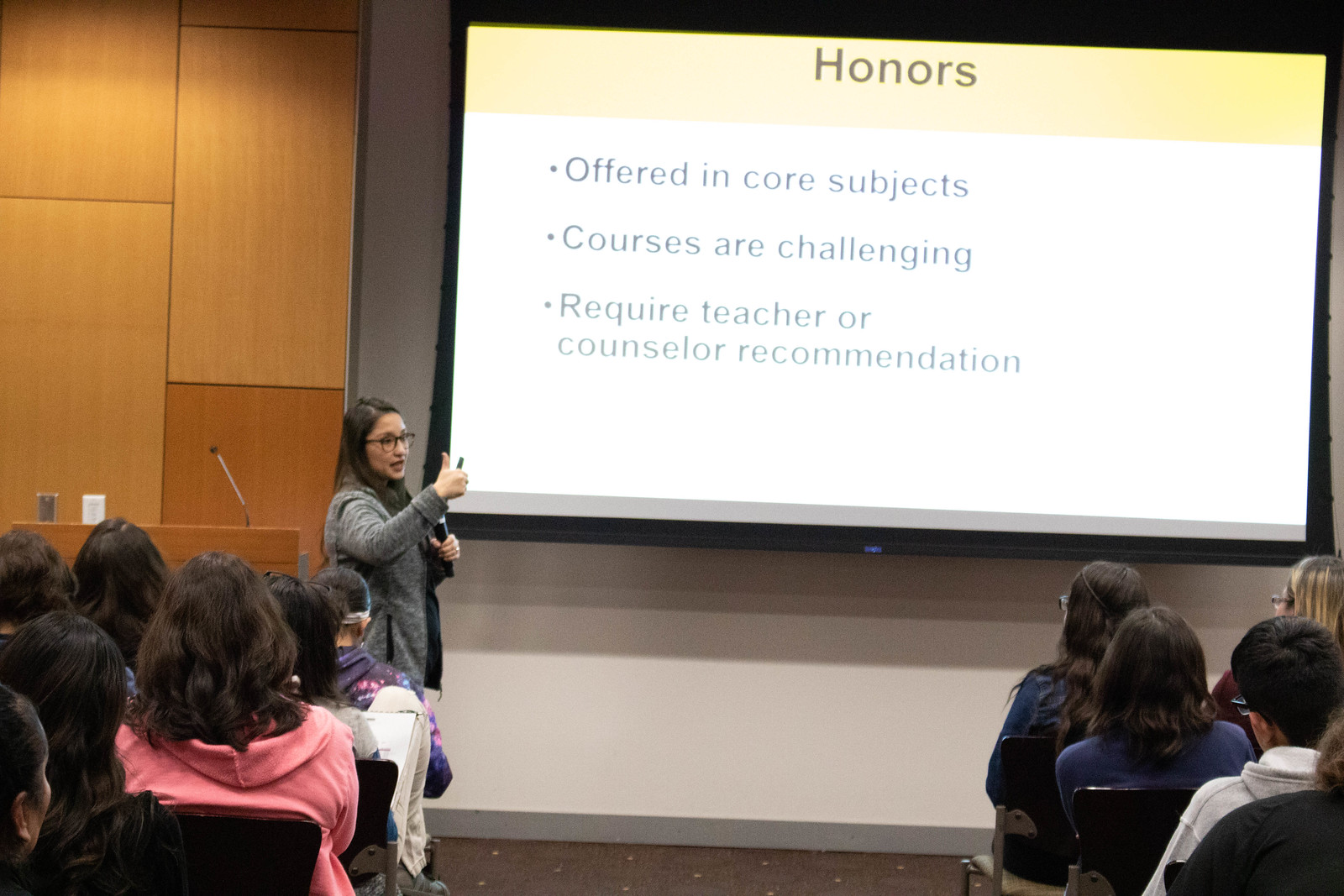In the image, a woman, possibly a teacher, is giving a presentation in a room filled with seated attendees. She has long brown hair, wears glasses, and is dressed in a gray long-sleeve jacket. She holds a clicker in her right hand and a microphone in her left hand. The screen behind her has a yellow and white background with a yellow header that reads "Honors." Under this header, there are three bullet points: "Offered in-course subjects," "Courses are challenging," and "Requires teacher or counselor recommendation." The seating is divided into two groups, with attendees on both the left and right sides, and a central aisle in between. Visible behind the presenter is a wooden podium with an attached microphone and a wooden backdrop. The image is shot from the back, showing the audience facing the screen with only the backs of their heads visible.